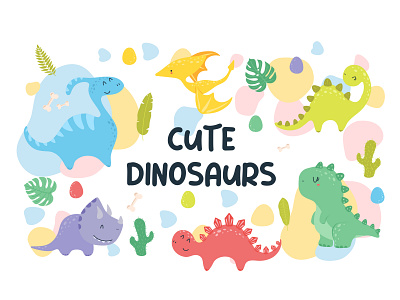This vibrant and playful illustration features a variety of cartoon dinosaurs, all set against a crisp white background. The center of the image is adorned with black, hand-drawn text that reads "Cute Dinosaurs," adding a whimsical touch to the scene. The dinosaurs, each with distinct colors and cheerful expressions, are scattered across the image. Notably, there is a friendly blue dinosaur and a gray triceratops positioned in the lower left corner. A joyful pink stegosaurus occupies the bottom area, while a yellow flying dinosaur hovers near the top. Accentuating their charm, the dinosaurs have black, hand-drawn eyes and facial features. The background is sprinkled with colorful blobs, green fern branches, a cactus, and a green feather, enhancing the overall lively and enchanting feel of the composition.